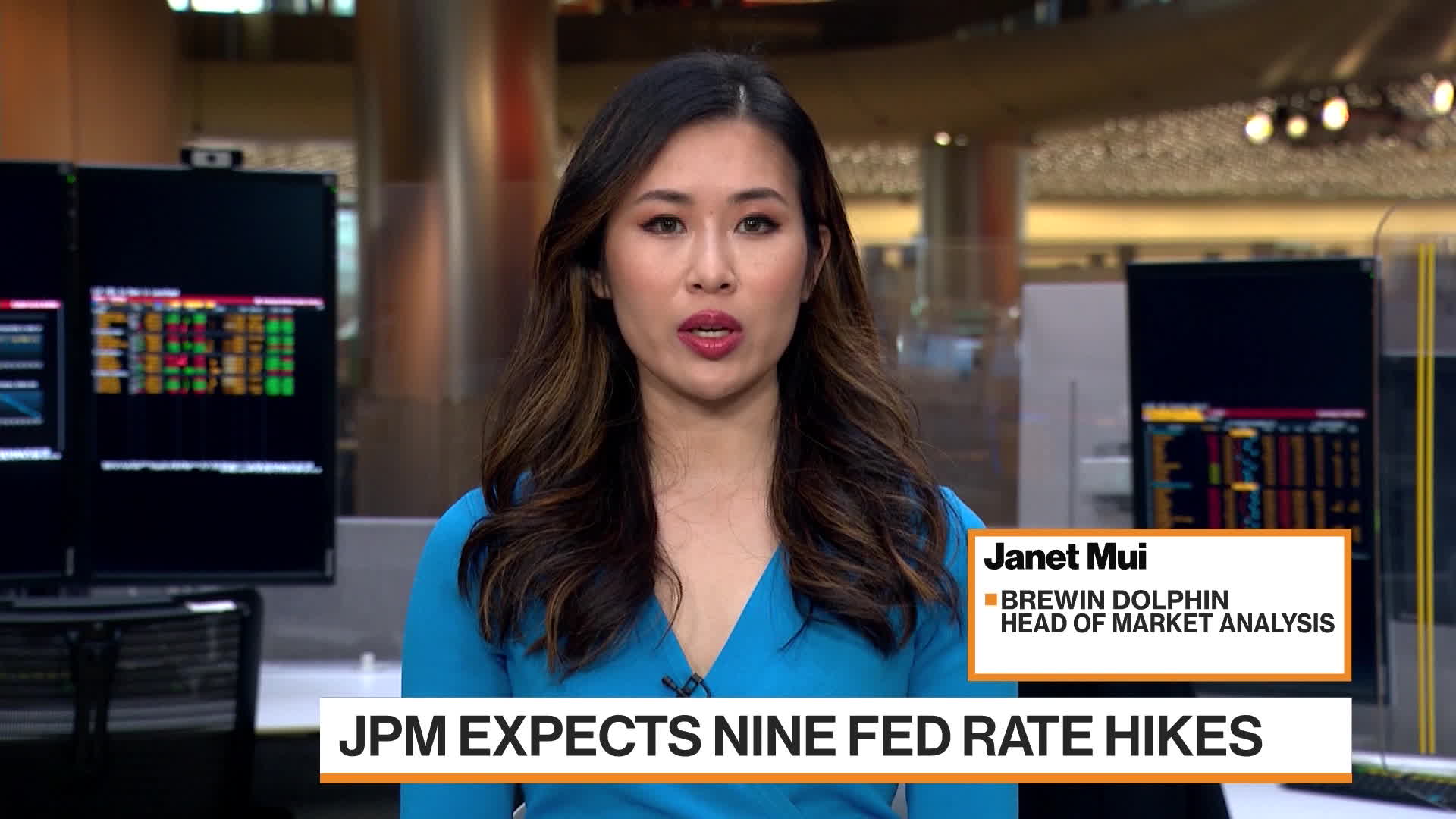This image captures Janet Mui, an Asian newscaster, in the midst of delivering a report. She is wearing a blue v-neck blouse with a microphone clipped at the bottom of the V. Her hair, a mix of light and dark brown with highlights, falls slightly longer than her shoulders and is parted to the side. Janet is staring straight ahead into the camera, her mouth slightly open mid-sentence, and her lips adorned with pink lipstick. The scene is a likely screen grab from a TV news broadcast, set against a background of multiple monitors displaying various statistics and a large rectangular window with two illuminated lights hanging above it. To her left and right are additional screens, adding depth to the room's technological ambiance. Overlaying the image is a text banner, with a white box bordered in orange that reads "Janet Mui, Bruin Dolphin Head of Market Analysis" in black letters. Directly below this, a white bar with black text states, "JPM expects nine Fed rate hikes." Janet Mui stands centered in the frame, clearly the focal point of the broadcast.